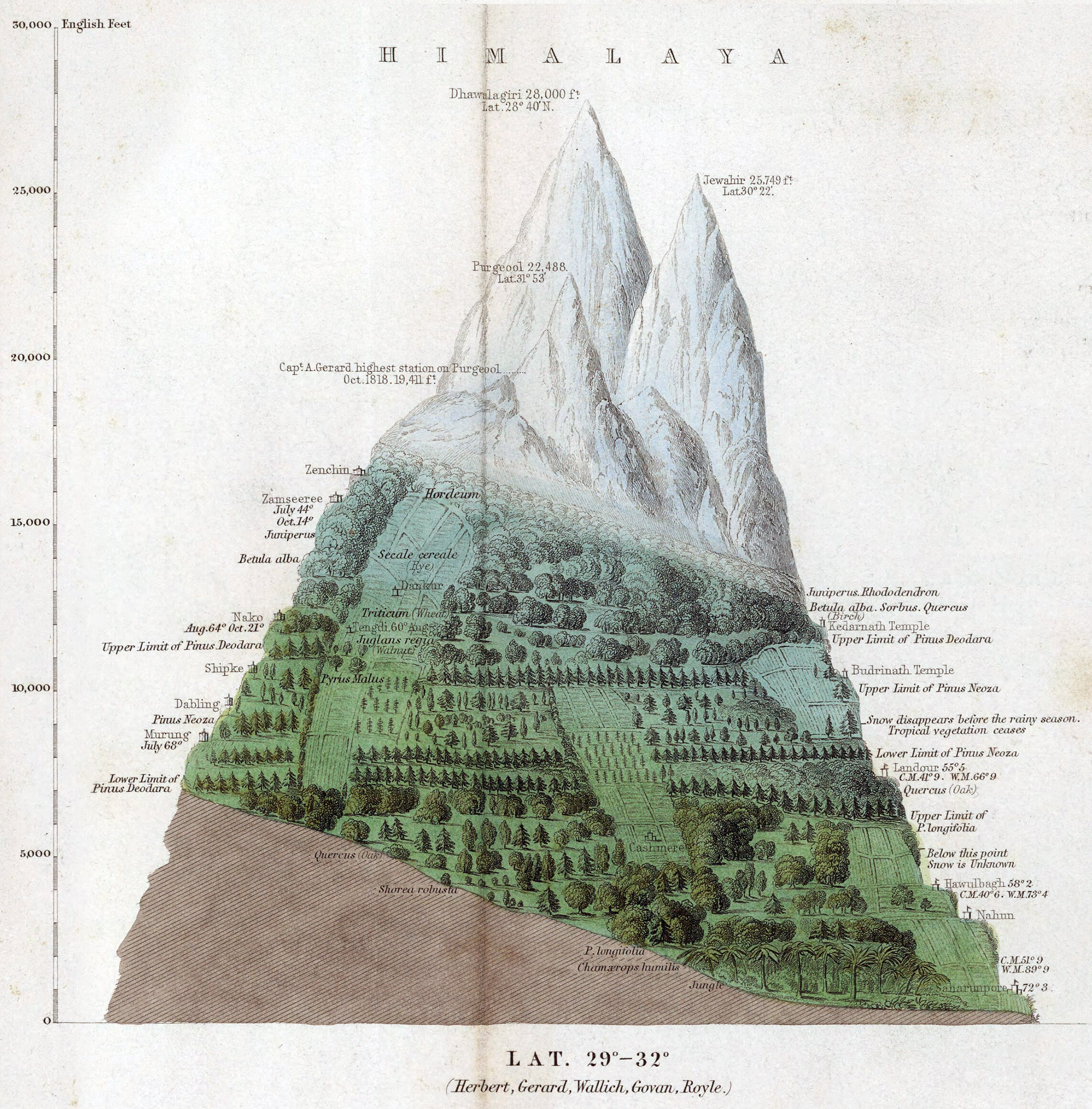This image is a detailed educational illustration of the Himalayan mountains, resembling an old map or textbook page. At the top, it prominently features the word "Himalaya." The illustration is vertically segmented with various elevations marked on the left side, descending from 30,000 feet to 5,000 feet. The peaks of the mountains are white, likely indicating snow, then transition into two shades of green symbolizing different vegetation zones, with distinct rows of trees including palms and pines, before tapering off into a brown base, representing dirt or lower altitudes. Additionally, the caption at the bottom lists latitudinal coordinates "LAT 29°-32°" and names such as Herbert, Gerard, Wallach, Gowan, and Royal, possibly denoting contributors to the map or study. The overall appearance suggests it's designed for educational purposes, providing detailed geographical and botanical information about the Himalayan region.